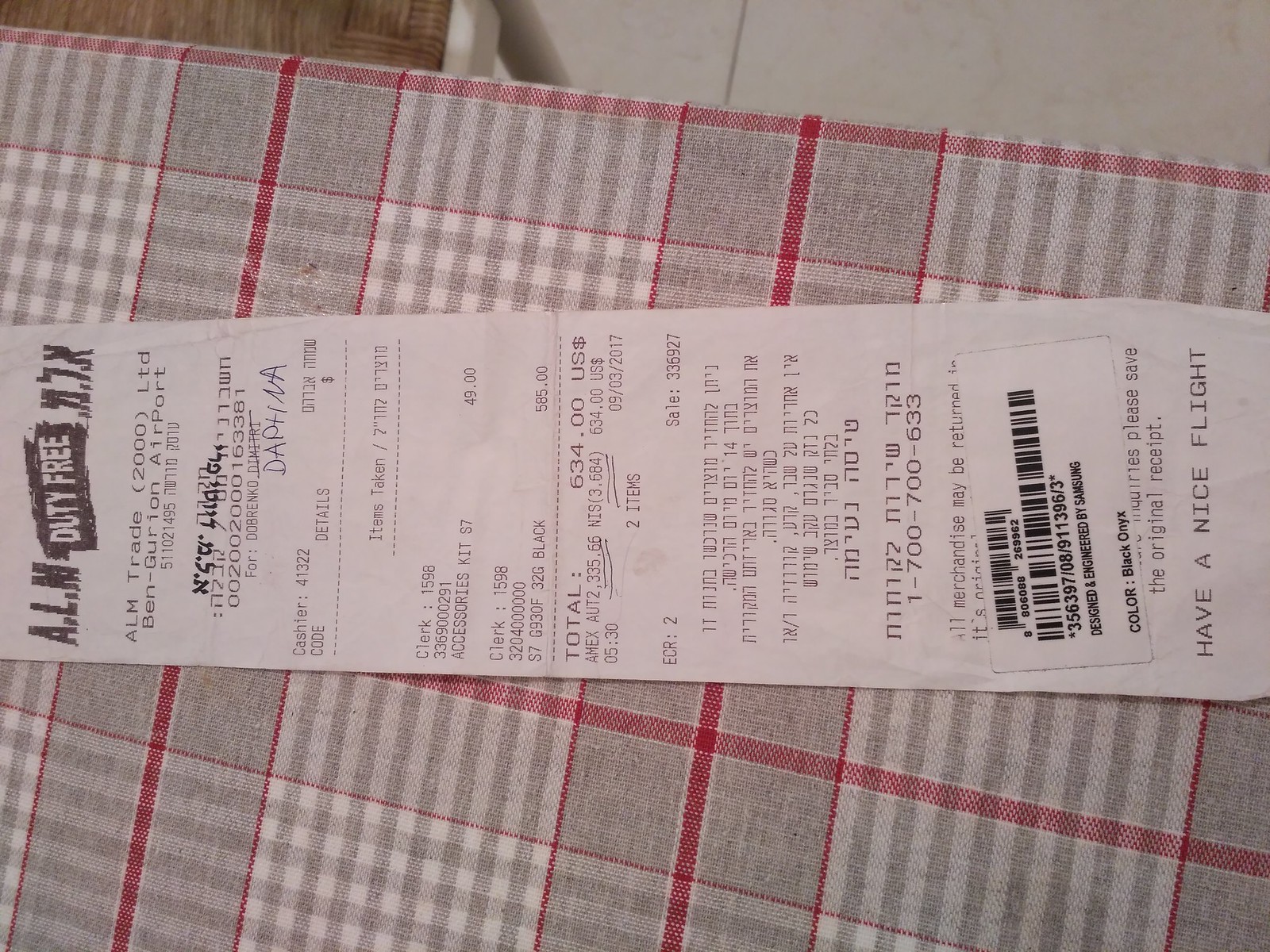The photograph showcases a receipt from ALM Duty Free, positioned horizontally on a gingham-patterned tablecloth. The tablecloth features a mix of light gray, white, and dark red stripes, forming a plaid pattern with certain areas appearing darker where the stripes intersect. The receipt, in black and white print, includes the header "ALM Duty Free" along with partially legible letters "N7X" and "Ben Gurion Airport." The itemized purchase on the receipt totals $634, broken down into an accessories kit priced at $49 and 32 grams of another item costing $585. Near the bottom, there is a foreign script and a sticker with a barcode. The receipt ends with the phrase "Have a nice flight." Additionally, there's a handwritten note on it, "DAFNA" in capital letters.